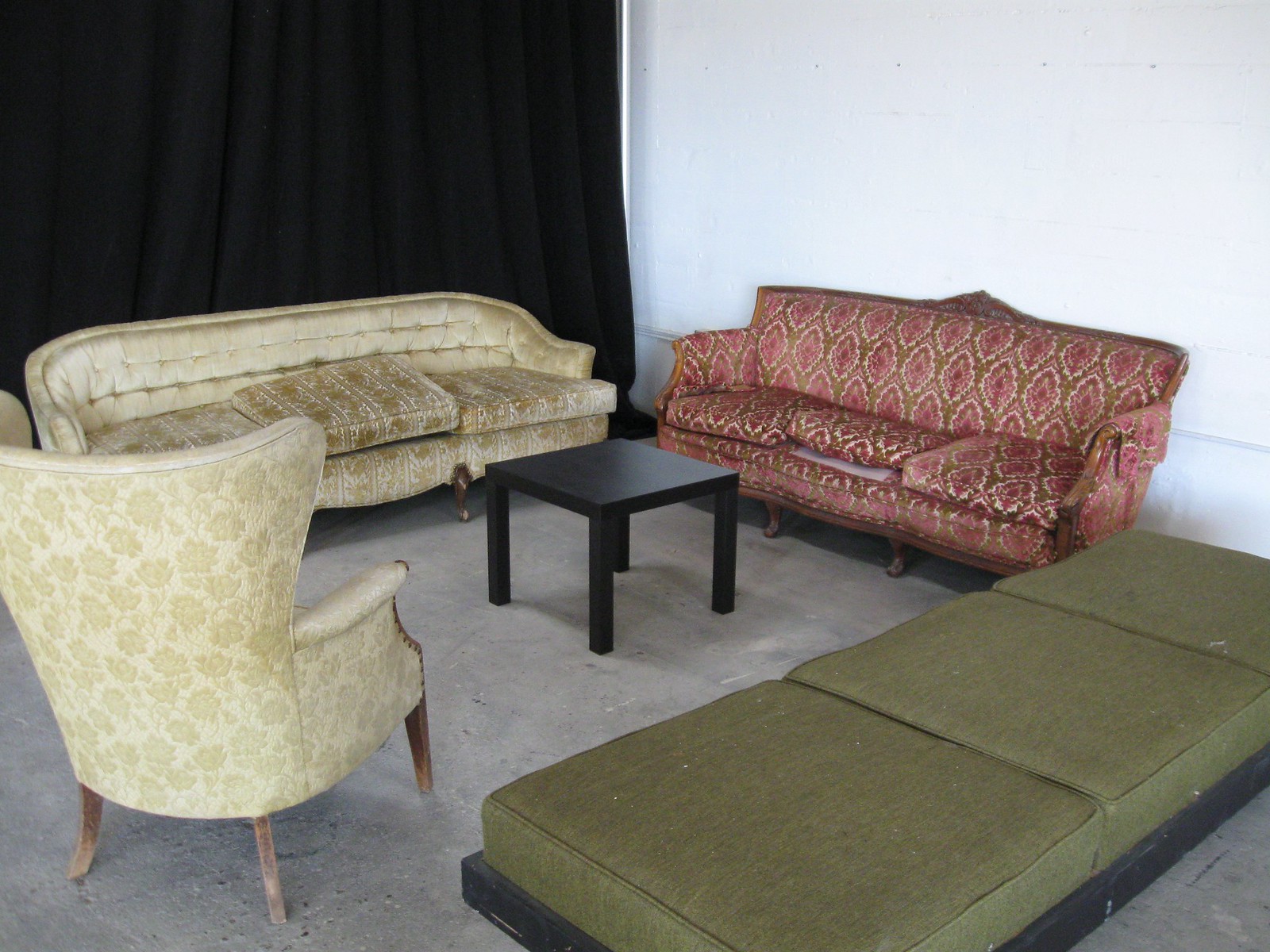The image is a color photograph of an eclectic interior room featuring a mix of vintage and mismatched furniture. The right wall is painted white, while the left side of the room is dominated by a floor-to-ceiling black draped curtain. The floor appears to have a worn wall-to-wall gray carpet.

Against the white wall, there is an ornately carved antique Victorian-style sofa with a wooden frame. The upholstery is a shabby burgundy with gold brocade pattern, and the raised center seat cushion reveals some white padding underneath. In front of the black curtain, there is a mid-century-style gold or champagne-colored velvet sofa with a tufted back and cloth feet.

In the lower left corner of the image, there's a classic wingback chair with a light cream and green floral pattern upholstery. The wooden legs of the chair are visibly scratched and in need of refinishing. Positioned centrally among the furniture is a simple, modern black Parsons coffee table that contrasts with its surroundings.

To the lower right side of the image, there is a low bench or daybed with three olive green cushions, suggesting a mid-century design without a backrest. All these pieces of furniture are set against the backdrop of the room, creating a staged yet intimate seating area.

The overall scene captures an interesting mix of old-fashioned elegance and stark modern simplicity, providing a striking visual contrast.